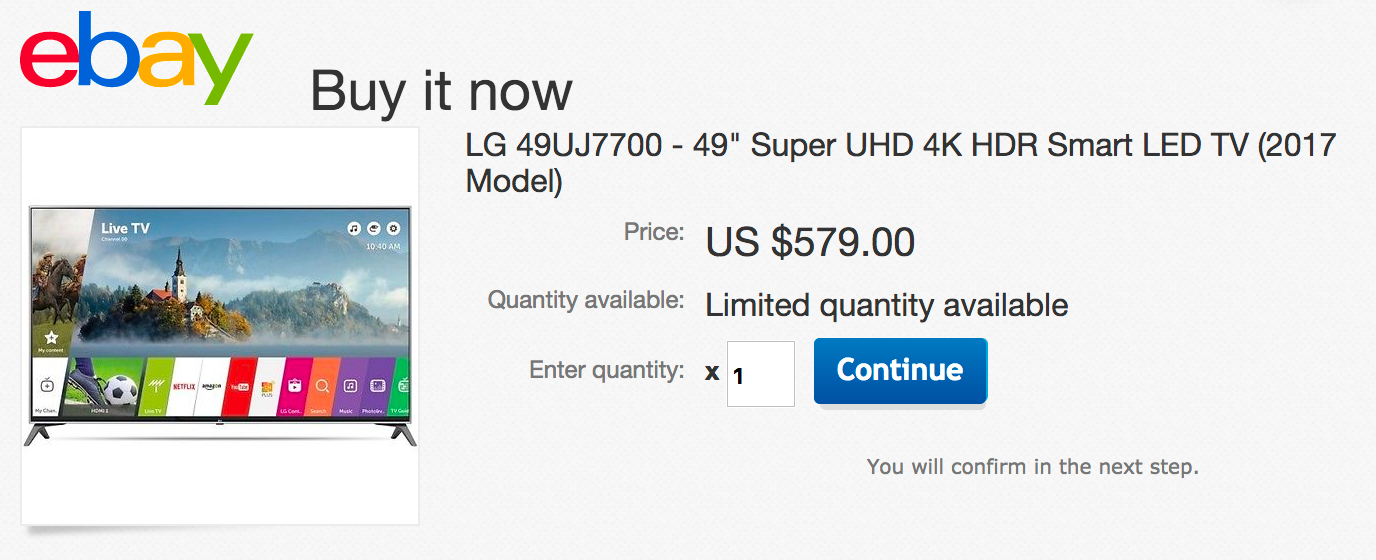This detailed eBay pop-up menu screenshot showcases a horizontal gray rectangle interface. Positioned in the upper left corner is the iconic eBay logo, featuring multicolored letters reminiscent of the Google logo. To the right of the logo, in bold black font, is the "Buy It Now" option.

Beneath this section, there's a high-resolution thumbnail image of a sleek flat-screen television set. The TV is a modern smart LED TV, displayed against a clean white background. Adjacent to the TV image, text in black font specifies the product details: "LG 49UJ7700-49 Super UHD 4K HDR Smart LED TV 2017 Model."

Directly below the product name, the price is listed in a combination of gray and black fonts: "Price: US $579." The scarcity of the item is emphasized with the phrase "Limited quantity available" printed in gray. A quantity selection field follows, containing an input box pre-filled with a "1" and a blue "Continue" button in white font.